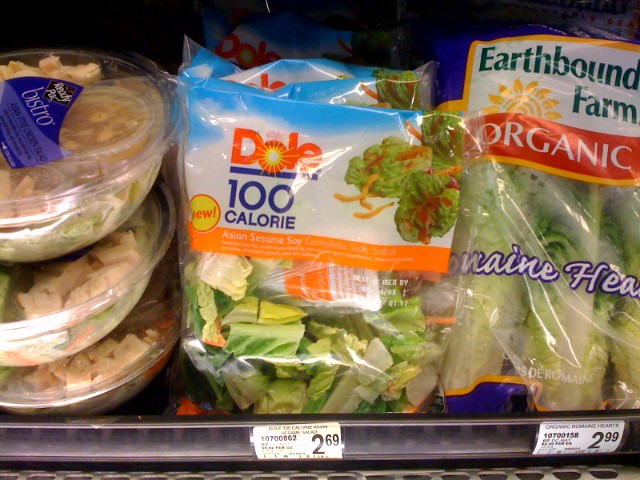A small section of a refrigerated shelf in a supermarket displays three salad-related products. On the left, there are three stacked ready-to-eat salad bowls containing mixed greens and pieces of chicken, accompanied by a small pot of dressing. In the middle, a bag of Dole salad features plain lettuce with a bit of shredded carrot, boasting 100 calories and priced at $2.69. On the right, a pack of organic romaine hearts from Earthbound Organic Farm contains approximately three hearts of lettuce and is priced at $2.99.